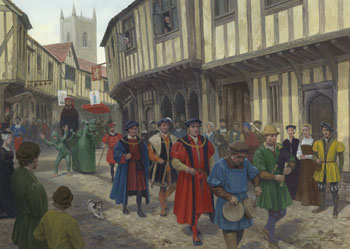This detailed painting appears to be a depiction of a historical celebration or parade, potentially set in the 17th or 18th century, though it could be earlier. The scene is set on a wide dirt road or alleyway, lined with brown and tan buildings on both sides. People are dressed in elaborate, oversized vintage attire, featuring muted yet vibrant hues of reds, blues, greens, yellows, browns, and tans. These individuals are part of a procession down the middle of the road, with onlookers standing on either side, suggesting a festive or significant event. In the far left distance, a castle head is visible, adding to the historical ambiance. The painting's overall muted color palette and detailed portrayal of period clothing hint at a celebration from a bygone era, possibly an interpretation seen in art or inspired by video game aesthetics.